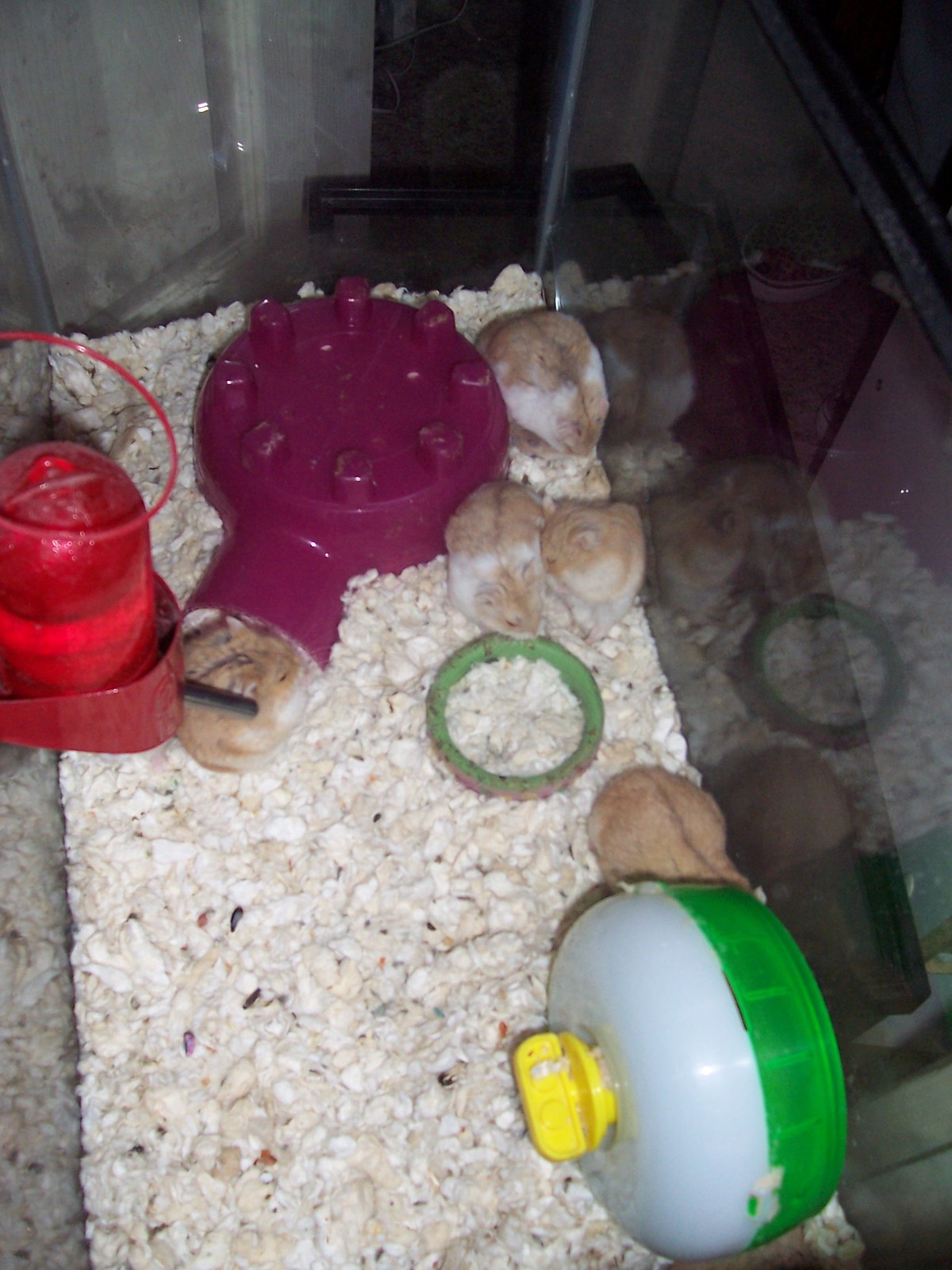This photograph captures an overhead view into a rectangular glass enclosure, resembling an aquarium, but designed for small rodents, likely hamsters. The base is covered with white, fluffy bedding material. In the bottom right corner, a green and white plastic hamster wheel with a yellow knob is positioned, partially occupied by one of the five brownish hamsters with greyish-white stripes. Centrally located in the cage is a green food bowl. At the top of the image, a purple plastic hideout with an entrance hole allows the hamsters to sleep inside. The left side of the cage features a red water dispenser with a spigot. The hamsters are scattered around the enclosure – one notably larger hamster is in the upper right corner atop a smaller one, while two are side by side below that pair. Each element within the cage provides a variety of activities and necessities for the hamsters, including hiding spots, feeding areas, and hydration sources.